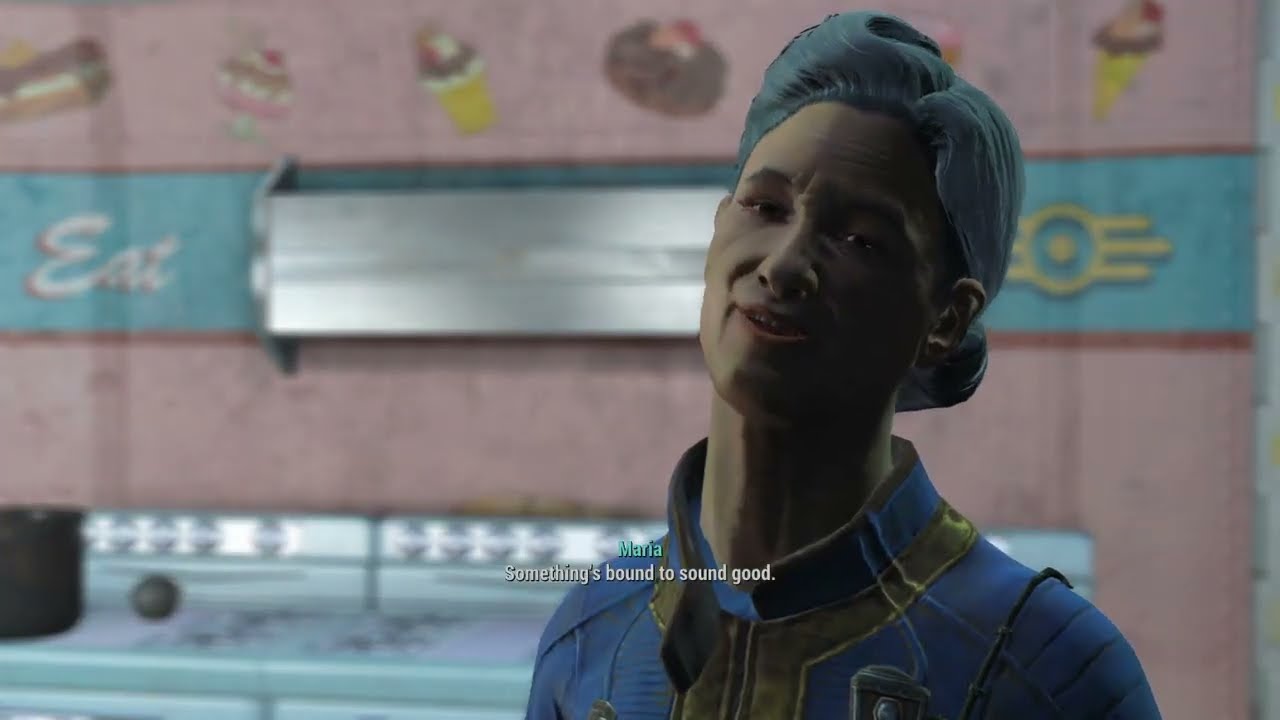The image is a screenshot from a video game, depicting an elderly character named Maria, who appears to be in her 60s. Maria has gray-blue hair styled in a pinup fashion and wears a blue jacket with gold trim, resembling a uniform. She stands in front of a pink, 1950s diner-like kitchen background. The backdrop includes symbols of desserts and ice cream snacks, a blue horizontal sign with the word "EAT," and a metallic shelf mounted above waist-high chest freezers and light blue stoves. Maria is speaking, with text at the bottom of the image that reads, "Maria: Something's bound to sound good." The scene suggests that Maria, possibly a cook, is offering a recommendation for something to eat.